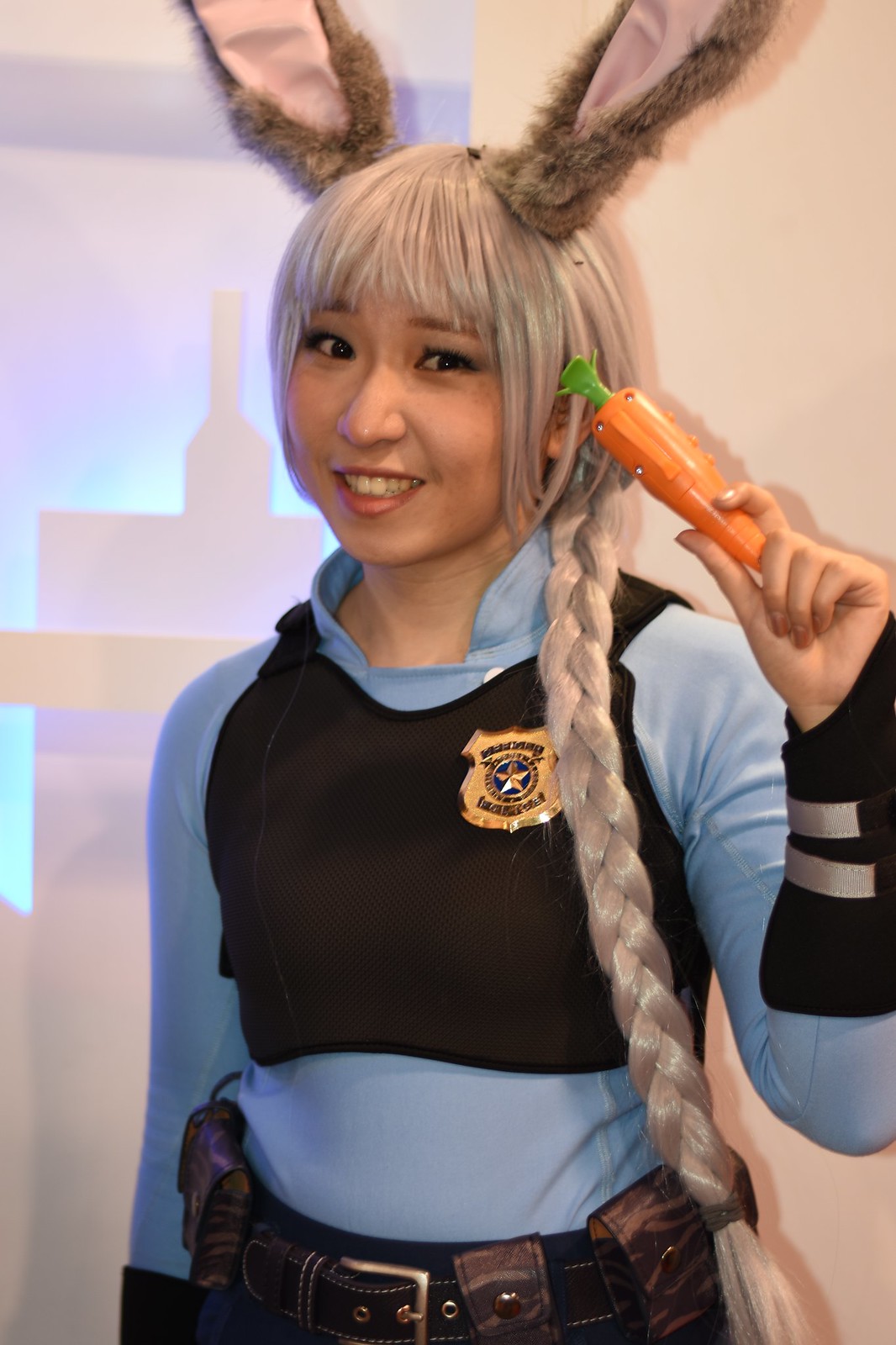The photograph features an Asian woman standing and facing the camera in what appears to be a cosplay outfit. She has deep blonde hair intricately braided into an extremely long ponytail that hangs down her right side, reaching below her waist. She wears a light blue, tight-fitted shirt with long sleeves, accented by a black cropped vest adorned with a large gold police badge featuring a star in its center. On her head, she sports a pair of bunny ears that are brown with pink interiors.

Her attire also includes a belt decorated with various pockets, suggesting a utilitarian function, and possibly a gun holstered to the side. The image captures her from the waist up, revealing the top of her blue pants. Her right hand is raised, holding a toy carrot with visible screws, colored orange with a green top. She is grinning, her teeth visible.

The photograph appears to have been taken indoors with frontal lighting that creates shadows in the background, which shows reflections in various shades of tan and blue, indicating some light source off-camera.